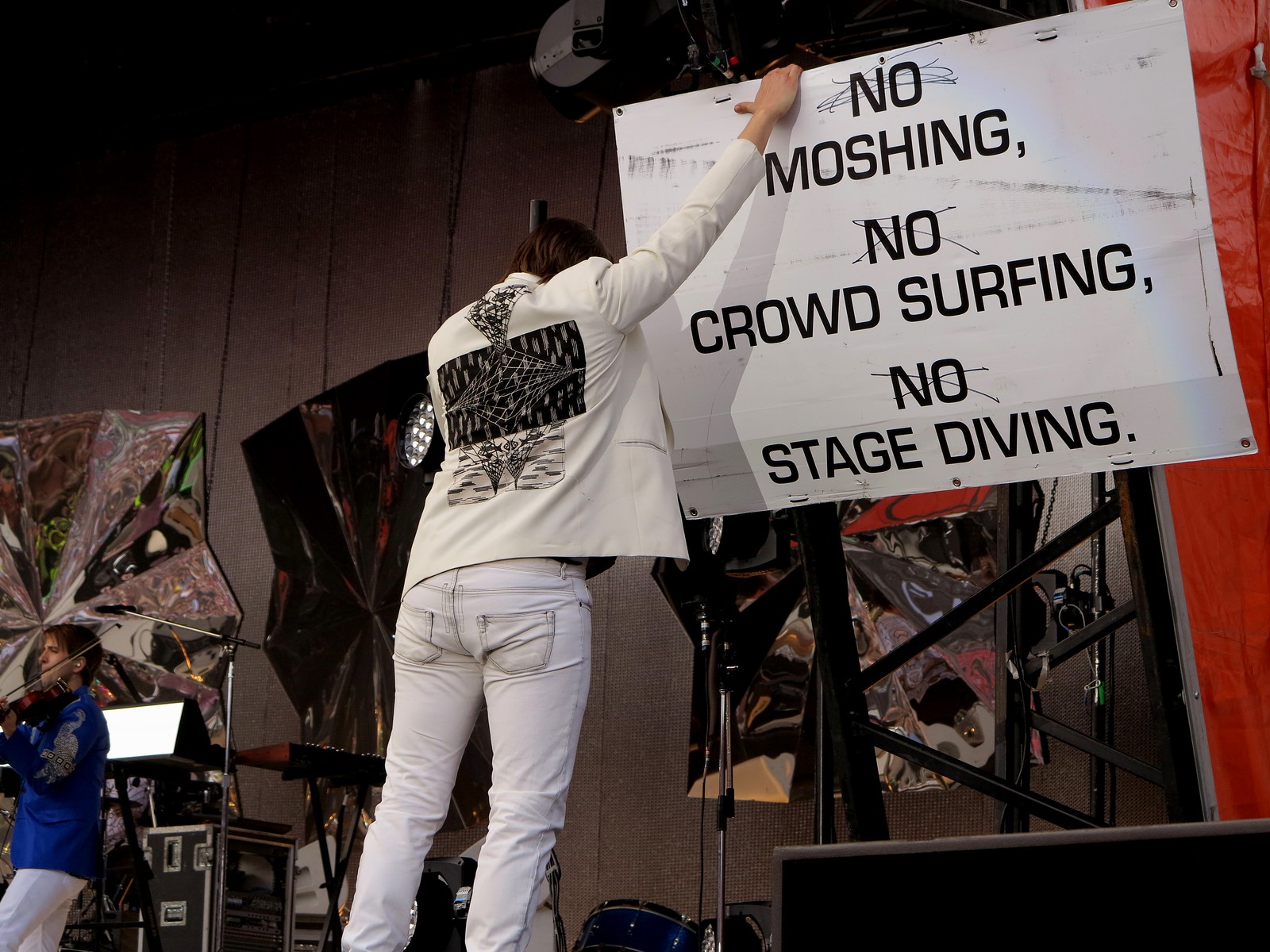This image captures a scene where a woman is setting up a stage, facing away from the camera. She is wearing a white suit jacket featuring a black artistic design on the back, paired with faded, nearly white blue jeans. She is in the process of putting up a sign with a white background and black uppercase letters, each centered on separate rows. The sign reads:

```
NO MOSHING

NO CROWD SURFING,

NO STAGE DIVING
```

However, it appears that someone has attempted to cross out the word "NO" in all three directives with a pen, making it look as though the sign permits moshing, crowd surfing, and stage diving. The background appears to be the backdrop of the stage, resembling a wooden structure or possibly a curtain.

To the left of the woman, another person, possibly a man, is seen. He is wearing a long-sleeve blue shirt and light blue jeans and is positioned facing towards the left side of the picture, allowing his face to be visible. This person is holding and playing a violin.